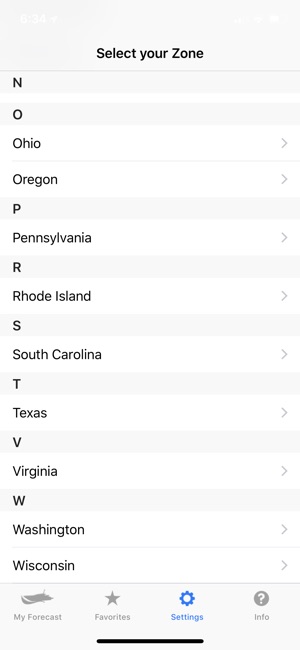The image showcases an interface for selecting geographic zones. At the top, a light gray header displays the text "Select Your Zone" in bold, black Arial font. Below, there is an alphabetized list of places, each segmented by letters. The letter "N" appears in bold on the left, followed by "O," both on gray backgrounds, while the overall background is white.

Under the letter "O," the options "Ohio" and "Oregon" are listed, each accompanied by a right-pointing gray arrowhead for further selection. These options are separated by a gray divider. The sequence continues with "Pennsylvania" under the letter "P," similarly denoted with a navigational arrowhead. Subsequent state listings include "Rhode Island," "South Carolina," "Texas," "Virginia," and "Washington." Another gray divider follows "Washington," indicating multiple listings and leading to "Wisconsin."

The footer, marginally smaller than the header, features a set of icons and labels. On the left, an indiscernible moon-like icon and a rectangular area are present, but the image's distortion makes them unclear. The text "My Forecast" appears in small gray lettering. Adjacent is a gray star labeled "Favorites," and to its right, a blue gear icon labeled "Settings," indicating its active selection. Further right, a circular icon filled with gray contains a bold white check mark, labeled "Info" in small gray text. Centered at the bottom, a dark gray line spans about one-third of the footer, suggesting a swipe-up gesture to exit the interface.